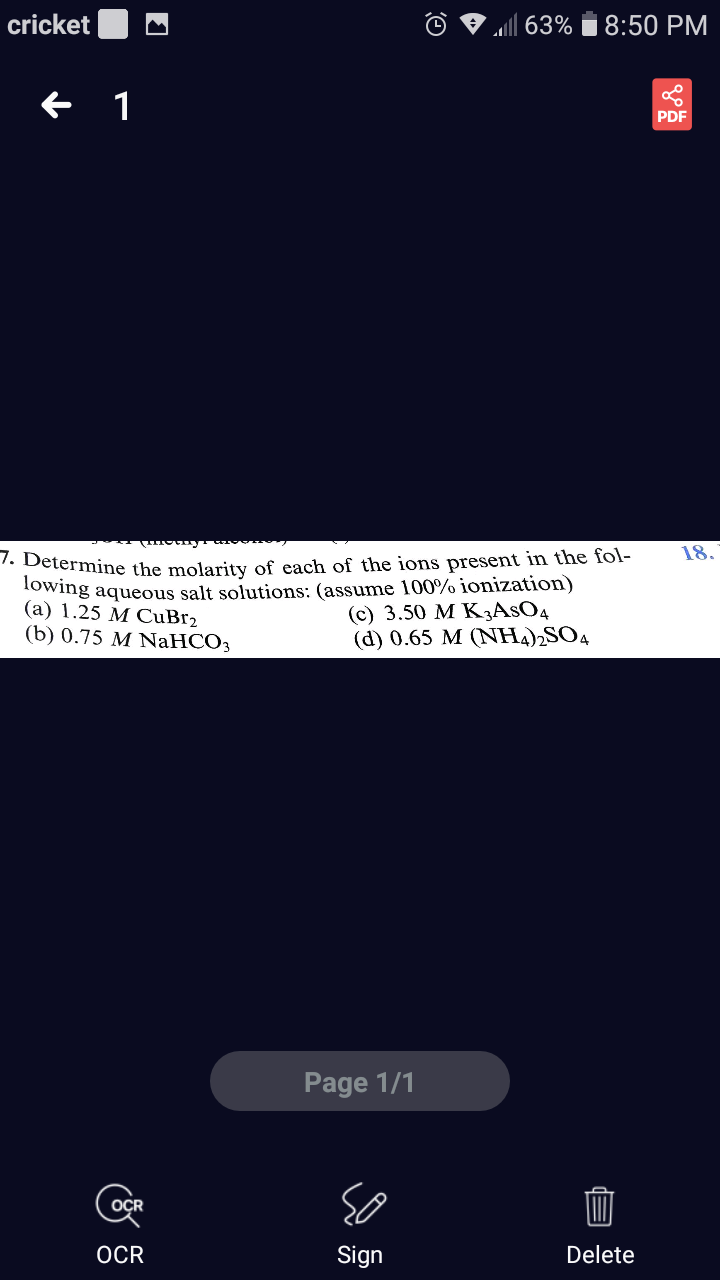The image features a predominantly black background with various details and elements arrayed across it. In the upper-left corner, the word "Cricket" is displayed in light gray font, accompanied by a light gray box adjacent to it. On the right side of the top row, the current battery level, "63%", is shown along with the time, "8:50 p.m."

Descending to the next row, there is a small arrow pointing to the left next to the number "1." To the right of this, there is a red box with the label "PDF" inside it.

Dominating the middle area of the image is a long horizontal box with a white background containing a word problem. The problem starts with "7." and reads, "Determine the molarity of each of the ions present in the following aqueous salt solution." Below this prompt, four multiple-choice options are neatly listed:
- A) 1.25 M \( CO_3 \)
- B) 0.75 M \( NaHCO_3 \)
- C) 3.50 M \( K^+ \)
- D) 0.65 M \( (NH_4)_2SO_4 \)

At the bottom of this word problem, it notes "Page 1-1" in reference. Along the very bottom of the image, three horizontal choices are presented: "OCR," "Sign In," and "Delete."